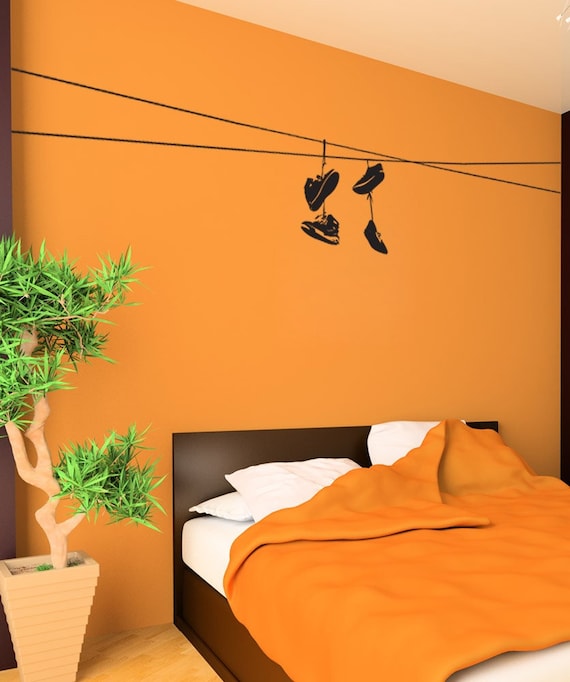The photograph depicts a distinctive and vibrant bedroom with a prominent bright orange wall that immediately catches the eye. Near the ceiling, two lines are painted horizontally across the wall, and from these lines hang two pairs of black sneakers—one pair of high tops and one regular—tied together in a manner reminiscent of shoes tossed over power lines. Below this intriguing feature is a spacious bed with a dark brown frame and headboard, which may be queen or king-sized. The bed is neatly made with stark white pillows and is covered by a burnt orange comforter, artfully folded into a triangle at one corner. To the left of the bed stands a large, lush green plant in a brown, triangular-shaped pot that adds a natural element to the room. The flooring is a mix of light and dark brown hues, creating a pleasing contrast with the vibrant walls and the dark, modern furniture.